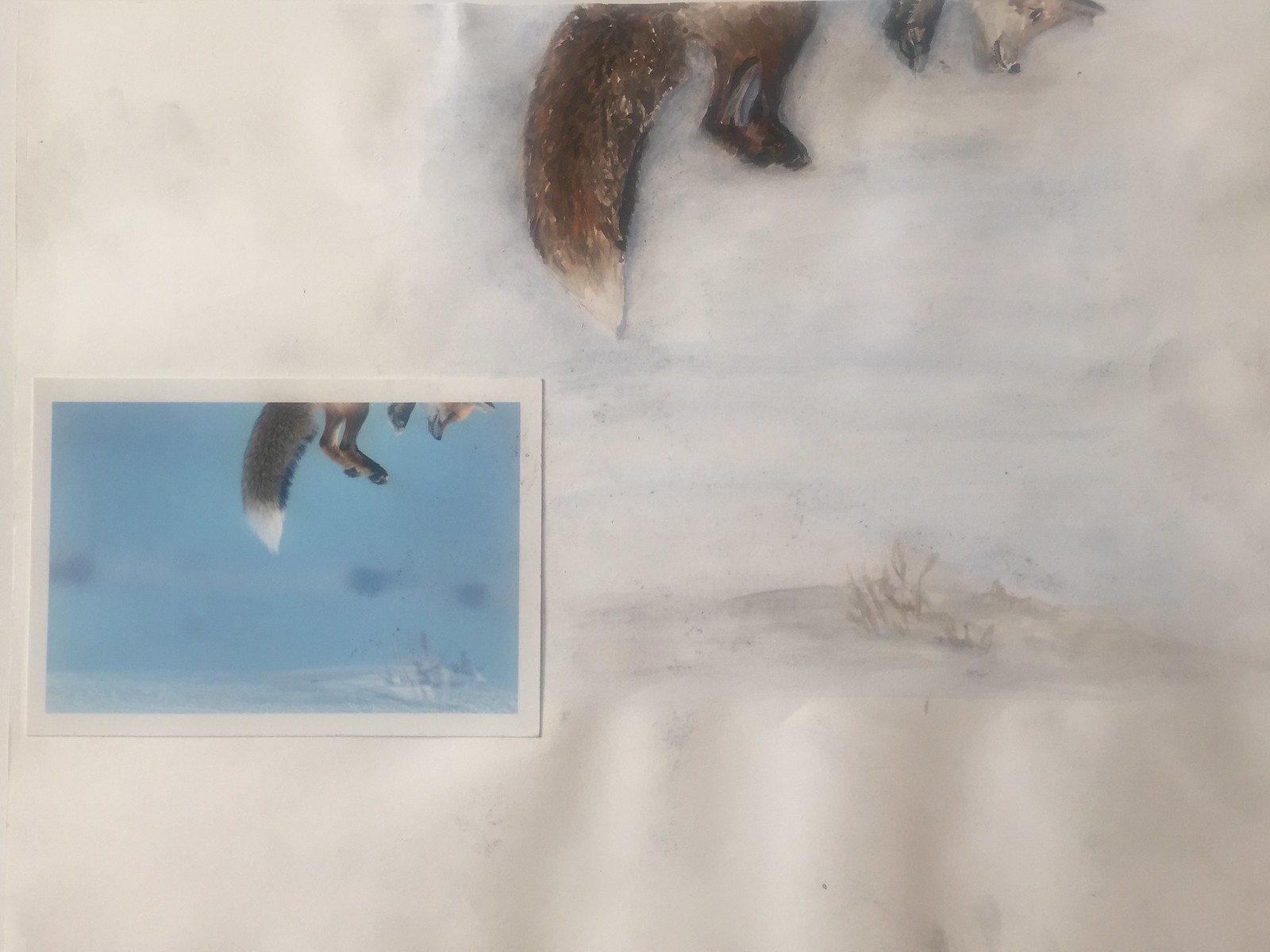This artwork captures the dynamic essence of a fox in mid-leap, set against an intriguing backdrop of slightly crumpled paper. The primary color palette of the background is a blend of soft whites and grays, accented by delicate sketches in bluish-gray tones. Dominating the upper center of the image is the vibrant, bushy tail of the fox, characterized by its rich brown hue and a distinctive white tip. Just beneath the tail, two black paws stretch out, adding to the sense of motion.

To the left side of the artwork, there is a smaller photograph that complements the main scene. This inset features the same energetic fox, but with a clearer emphasis on its motion. The background in this section is a muted blue, and it showcases the fox's tail, hind legs, and one front paw, each rendered in expressive detail. The image is cropped at the fox's nose, enhancing the impression that the fox is bounding out of the frame, perpetually frozen in the thrilling act of jumping.